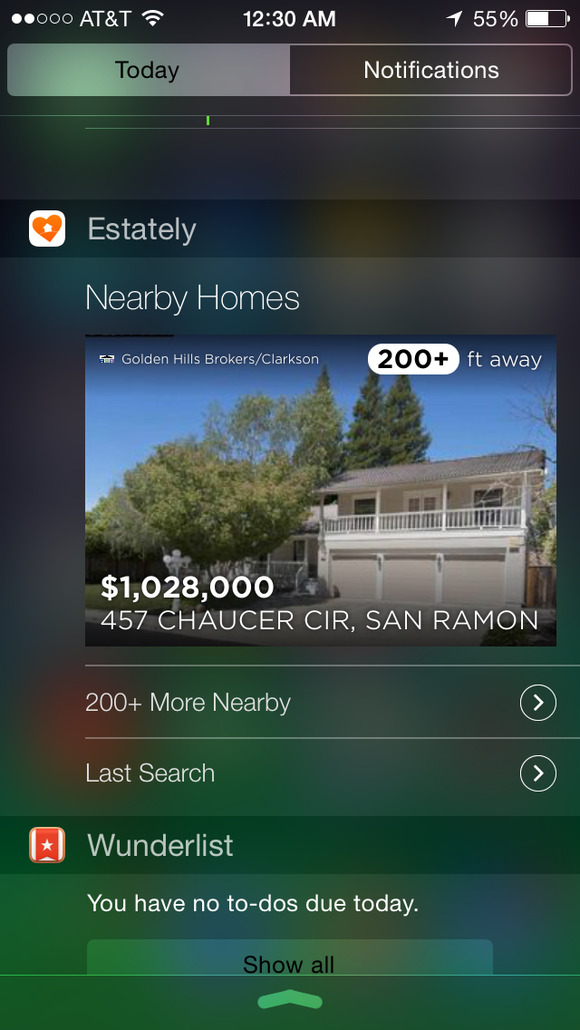Located at 457 Chaucer St., San Ramon, this majestic property is listed at $1,028,000. The house features a unique design with a robust structure built on top of three spacious garages. The exterior showcases a modern aesthetic with white railings, windows, and doors, complemented by a gray roof. A large cement pad in the front provides ample space for outdoor activities. The property is surrounded by lush greenery, including large trees, creating a serene environment. With proximity to local amenities and listed by Golden Hills Brokers, this home offers both luxury and convenience. Note: Notifications and app information irrelevant to the property have been excluded for clarity.